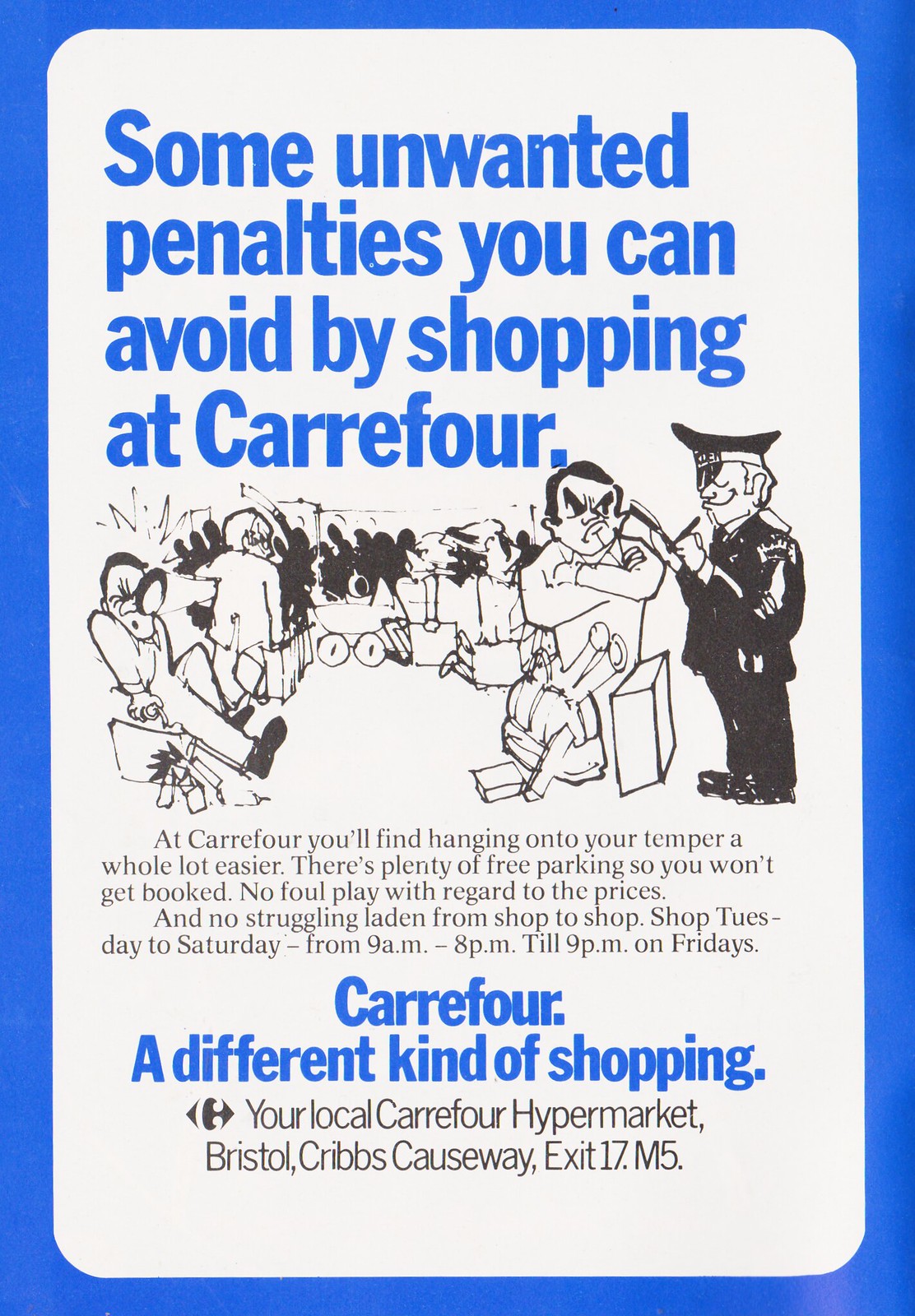This detailed advertisement from Carrefour features a vibrant poster set against a blue-bordered white background with prominent blue and black text. At its center, a drawing depicts a bustling scene, possibly an airport, where a policeman is writing a ticket to an angry traveler among a crowd. The ad conveys that by shopping at Carrefour, customers can avoid unwanted penalties. It emphasizes the benefits of shopping there, stating: "At Carrefour, you'll find hanging onto your temper a whole lot easier. There's plenty of free parking so you won't get booked. No foul play with regards to prices and no struggling laden from shop to shop." The text highlights their operating hours, "Tuesday to Saturday from 9 a.m. to 8 p.m., and until 9 p.m. on Fridays," and directs customers to the local Carrefour hypermarket at Bristol, Cribs Causeway, exit 17, M5, promoting it as "a different kind of shopping."